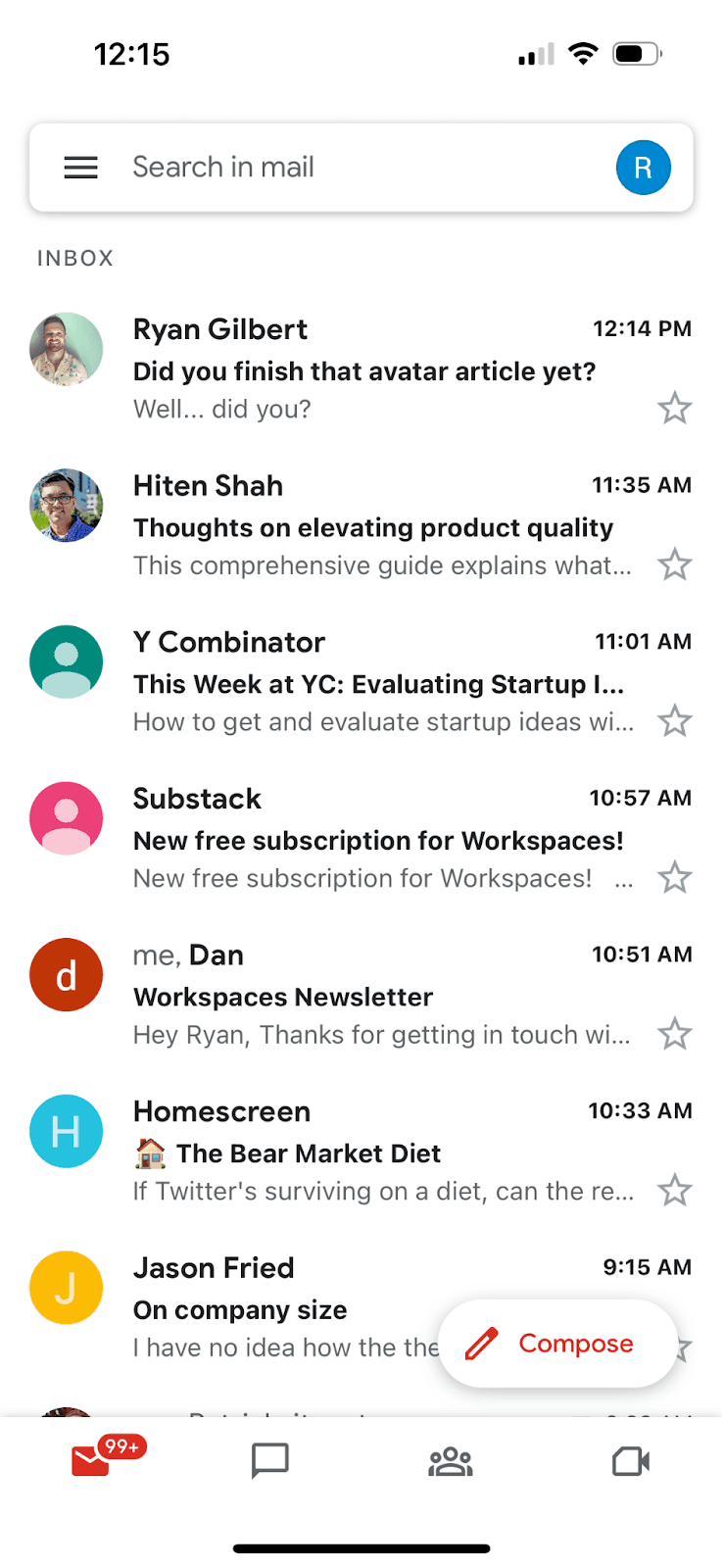The screenshot captures the interface of an email inbox from a cell phone. The upper left-hand corner features the time "12:15" in black text. Adjacent to the time, on the right, are three icons indicating signal strength, Wi-Fi connection, and battery status (the battery is approximately half-filled).

Below the status bar, a search box is prominently displayed. On the left side of this box are three horizontal lines, indicating a menu or navigation drawer. The text "Search in Mail" is centered within the box, and a small circle containing a white "R" occupies the right end of the box.

Under the search box, the word "Inbox" designates the current view, which displays a series of emails. There are eight emails visible in the screenshot, each featuring an avatar icon to the left and a snippet of text, sender information, and timestamp to the right.

1. The first email shows an avatar of a white male wearing a checkered shirt against a green background. The sender is "Ryan Gilbert" with the subject line, "Did you finish that Avatar Circle article yet? Well, did you?" The timestamp reads "12:14 PM."

2. The second email features a white male avatar wearing glasses and a blue shirt. The sender is "Hinton Shah" with the subject, "Thoughts on elevating product quality. This comprehensive guide explains what." The timestamp is "11:35 AM."

3. The third email displays a generic avatar against a green background, from "Y Combinator," with the subject line, "This week at YC evaluating startups." The email was received at "11:01 PM."

4. The fourth email has a generic red avatar and is from "Substack," with the subject, "New free subscription for workspaces." The timestamp reads "10:57 AM."

5. The fifth email features a red circle with a "D" and is from "Me, Dan," with the subject, "Workspace Newsletter." The email is timestamped "10:51 AM."

6. The sixth email is indicated by a blue circle with a capital "H." The sender is "Home Screen," and the subject is "The bear market diet." The time received is "10:31 AM."

7. The seventh email shows a yellow circle with a "J" and is from "J Fried," with a subject line, "Company size." The timestamp is "9:15 AM."

The visual elements and structure of the inbox provide a clear and organized view of the user's recent emails.